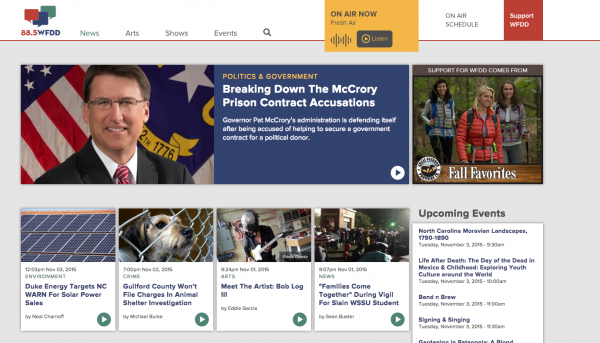The horizontally oriented screenshot captures the homepage of the 88.5 WFDD website. Dominating the upper section is the station’s distinctive red, green, and blue logo positioned in the top upper corner. To the right, a yellow box prominently displays the current broadcast with the text "On Air Now: Fresh Air," accompanied by a 'Listen' button located at the far right corner, inviting visitors to tune in live.

A white banner stretches across the top of the image, featuring links that read "On Air Schedule" and "Support WFDD." Notably, the screenshot spotlights the "Support WFDD" section in the center. Just below this banner, the header bar includes navigation options for "News," "Arts," "Shows," "Events," and a magnifying glass icon for search functionality.

The page’s main content is organized into articles and media. The top-left section showcases the leading article featuring a man smiling with flags in the background. The headline reads "Politics and Government: Breaking down the McCrory prison contract accusations," indicating a politically charged piece. This article also includes a small play button and is supplemented by four additional play areas beneath it, each linked to different videos.

On the top right-hand side of the webpage, a photograph captures three women enjoying a hike, labeled "Fall Favorites." Farther down, in the lower right-hand corner, a section titled "Upcoming Events" lists five clickable events, encouraging user engagement by redirecting to detailed event pages.

Overall, this detailed screenshot effectively highlights the multifaceted content and interactive elements available on the 88.5 WFDD website.